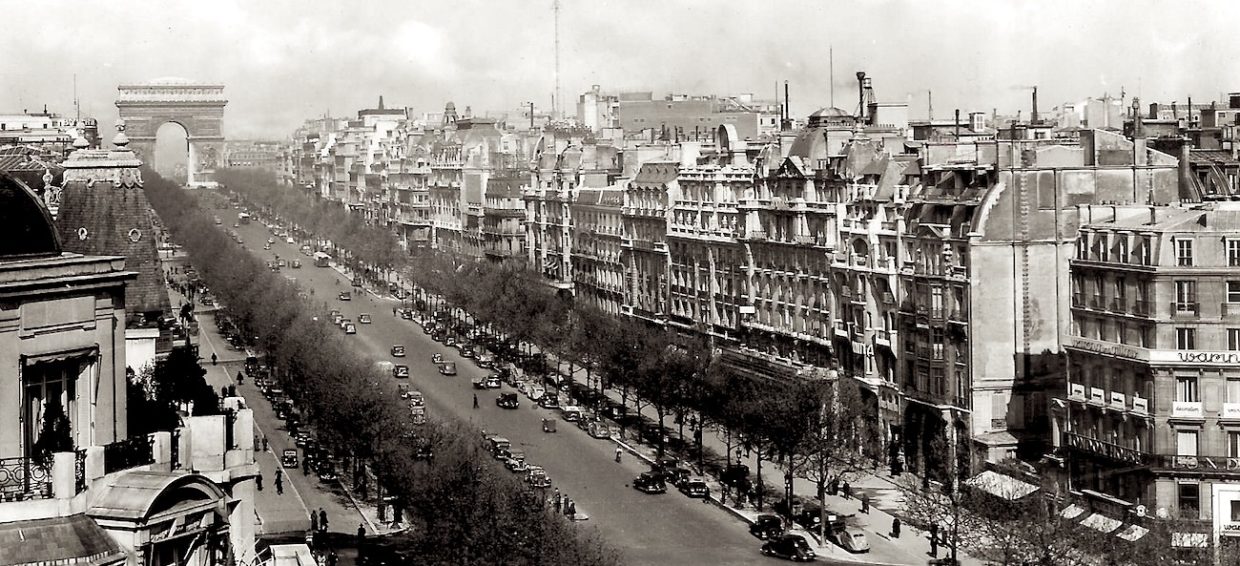This is a panoramic black and white photograph capturing a bustling cityscape, most likely Paris in the 1920s or 30s. The focal point of the image is the iconic Arc de Triomphe, standing magnificently at the end of a long, tree-lined avenue, which could very well be the Champs-Élysées. The street is alive with activity, featuring numerous old-fashioned cars reminiscent of Rolls-Royces, parked and driving along the road. On both sides of the avenue are tall, multi-story buildings, approximately four to five stories high, with shops on the ground level and apartments above. The photo appears to be taken from a rooftop, possibly around five or six stories high, providing a broad view of the city block below. Dense trees line the sidewalks, and there is a noticeable presence of people walking along the streets. In the distance, behind the monumental arch, the outline of what might be a factory or other industrial buildings can be seen against the very cloudy sky. The photograph captures the essence of early 20th-century Paris, with its characteristic architecture, bustling streets, and an air of historic charm.